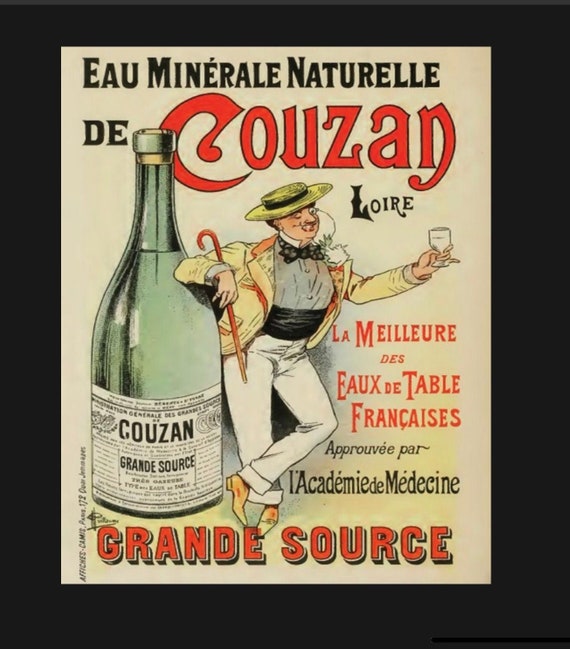This vintage advertisement for Kuzan features an intricate cartoon caricature of a debonair man leaning against a towering, green, wine-shaped bottle of Kuzan mineral water. The background of the image is tan with a black border, and the top reads "Au Mineral Naturel de Couzon" in elegant black lettering, while "Kuzan" is prominently displayed in bold red letters. The man in the image is stylishly dressed in a distinctive ensemble: a cream-colored jacket, a white brimmed straw hat, a black bow tie, white pants, and gold shoes. He sports a monocle and a black cummerbund, adding to his distinguished appearance. His right arm is outstretched, holding an empty brandy glass, and his left arm leans confidently against the bottle, where he also grips an orange cane. The bottle bears a white label that reads "Couzon Grand Source". Below, additional text in French mentions approval by the "Académie de Médecine" and reiterates in red, “Grand Source,” emphasizing the prestigious endorsement of this vintage mineral water.